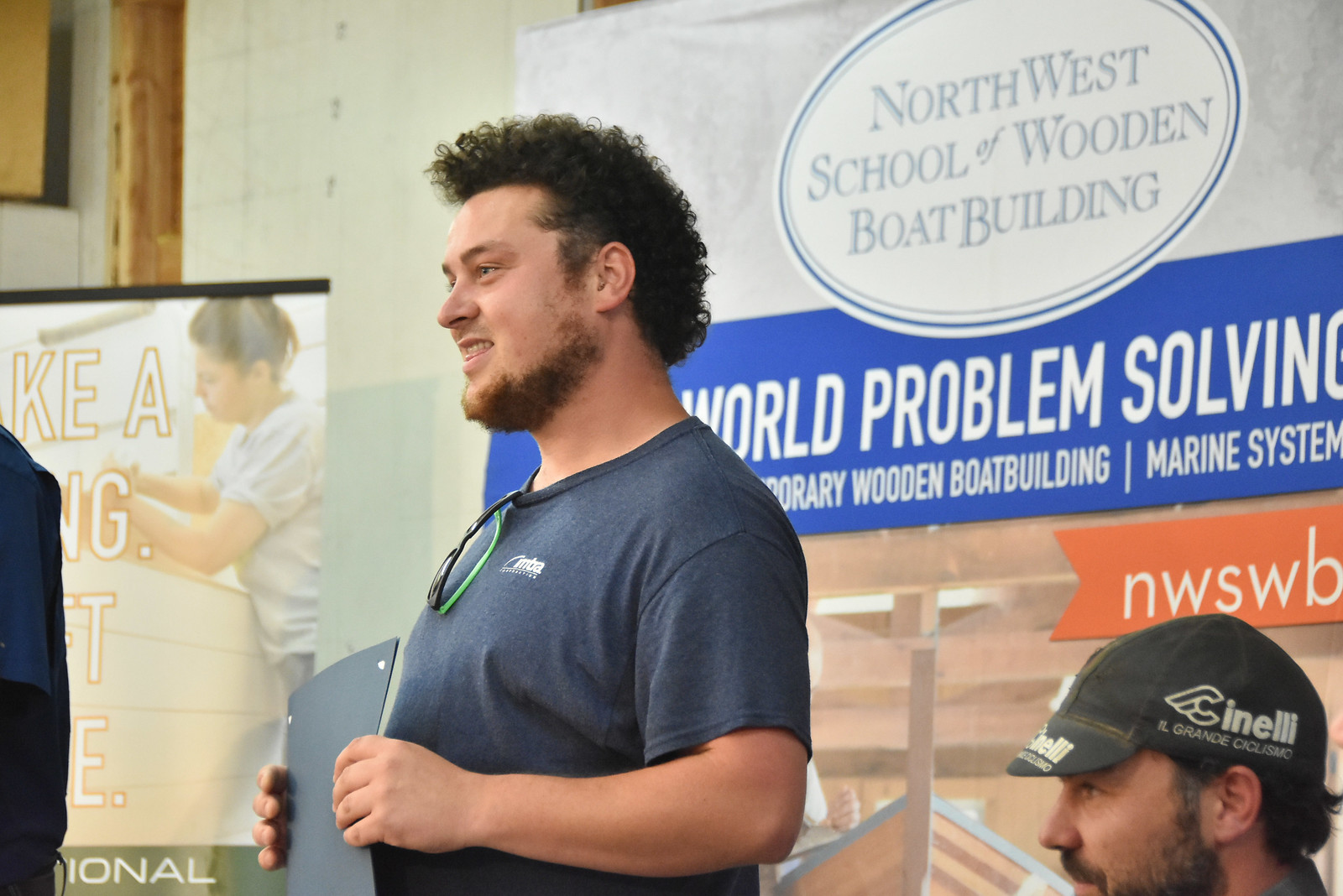This detailed color photograph, in landscape orientation, captures a scene on stage at the Northwest School of Wooden Boat Building. Central to the image is a man in his thirties, with brown hair and a beard, wearing a blue t-shirt. He stands slightly left of center, facing left, with a blue pamphlet held close to his chest. To his right and towards the bottom of the image is another man, wearing a white cap and sitting down, focused on the standing speaker. The background features a prominent poster displaying the school's name along with a blue stripe inscribed with "World Problem Solving" in white text, emphasizing their educational mission. The setting appears to be indoors, suggesting a midday event, with various posters and potential workshop slides partly visible, indicating an active and engaging environment dedicated to boat building craftsmanship.